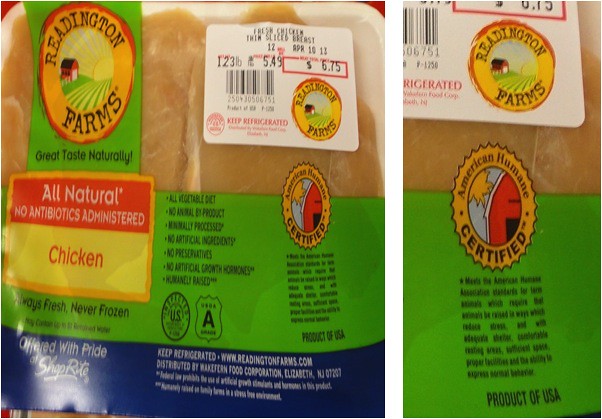This image features a side-by-side close-up of two photographs, with the left image being the focal point due to its larger size.

The main photograph showcases a pack of thin-sliced chicken breasts placed on a white Styrofoam tray and sealed with clear plastic wrap. The top section of the packaging is transparent, allowing an unobstructed view of the chicken. The remaining part of the packaging is adorned with a green and blue label from "Reddington Farms." The label prominently advertises the product as "All Natural" and "No Antibiotics Administered." Additional text assures buyers that the chicken is "Always Fresh, Never Frozen." Below these claims, the packaging lists various quality assurances such as "No Preservatives," "No Growth Hormones," and "No Animal Byproducts." The price is indicated at $5.49 per pound, with this specific tray costing $6.75.

The second, smaller photograph zooms in on the price tag of the same chicken package. It provides a closer look at the "American Humane Certified" label and includes a paragraph of text, though it is too blurry to read clearly.